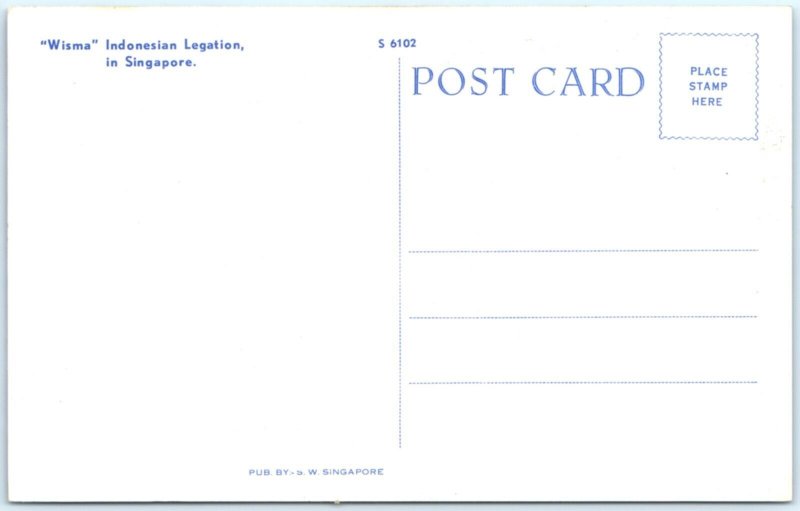This is the back of a blank postcard, primarily white with light blue writing and detailing. It features the label "WISMA Indonesian Legation in Singapore" on the left side, hinting this postcard is from Singapore. At the top center, there's an inventory number: S6102. There's also a blue printed label at the bottom that says "pub. by SW Singapore." The postcard's text is all in light blue. The right side prominently displays the word "POSTCARD" with three horizontal lines beneath it for the address. A square for the stamp is placed next to "POSTCARD." The card is divided down the middle by a line, separating the left half intended for a message from the right half designated for the address. The postcard has an overall framework of light blue, possibly reflecting the surface it's placed on in the image.